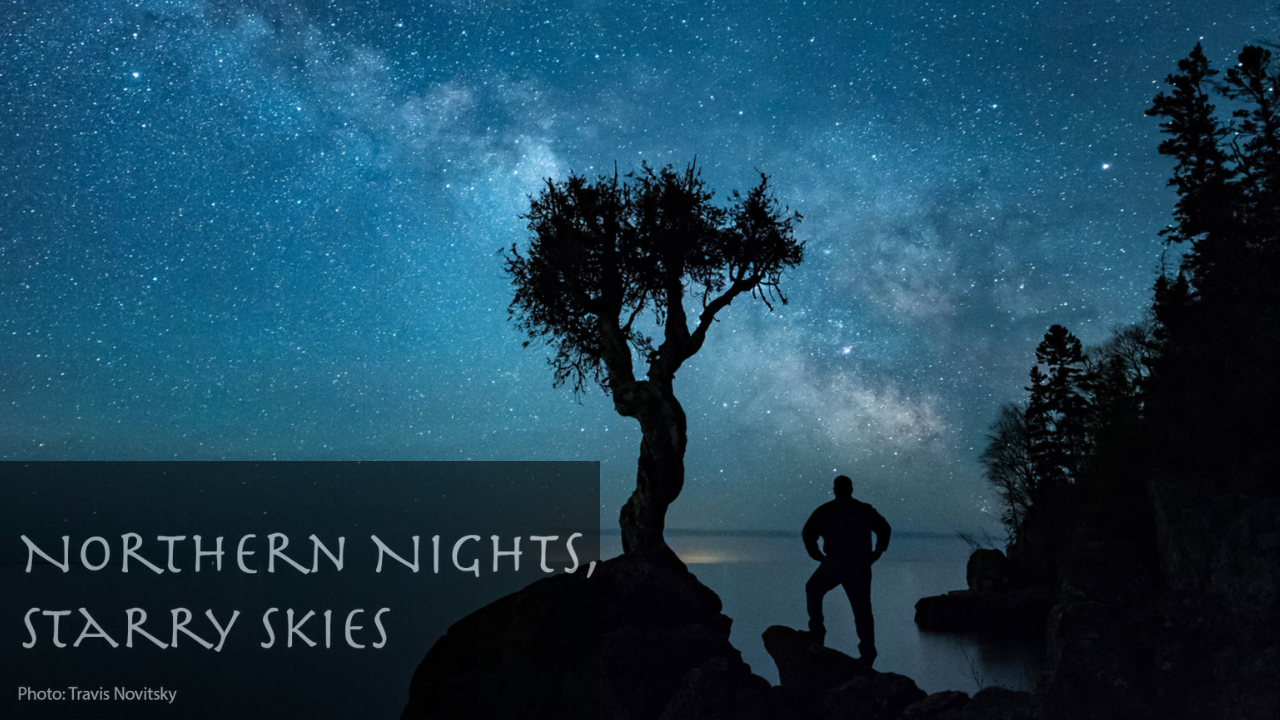In this captivating horizontal photograph, a dark blue night sky brimming with countless white stars stretches across the entire scene. Dominating the middle of the image is a twisted tree, silhouetted in black, with indistinguishable leaves or flowers. To the right, additional foliage appears in silhouette, contributing to the serene nocturnal tableau. A lone man stands poised on a rocky cliff, his hands on his hips, gazing wonderingly at the celestial display over what seems to be a lake or river, his figure also rendered as a silhouette. The bottom left corner of the image features a semi-transparent gray banner with bold white text that reads "NORTHERN NIGHTS STARRY SKIES," crediting "Photo Travis Nowitzki." The overall effect is a mesmerizing blend of natural beauty and artistic composition.